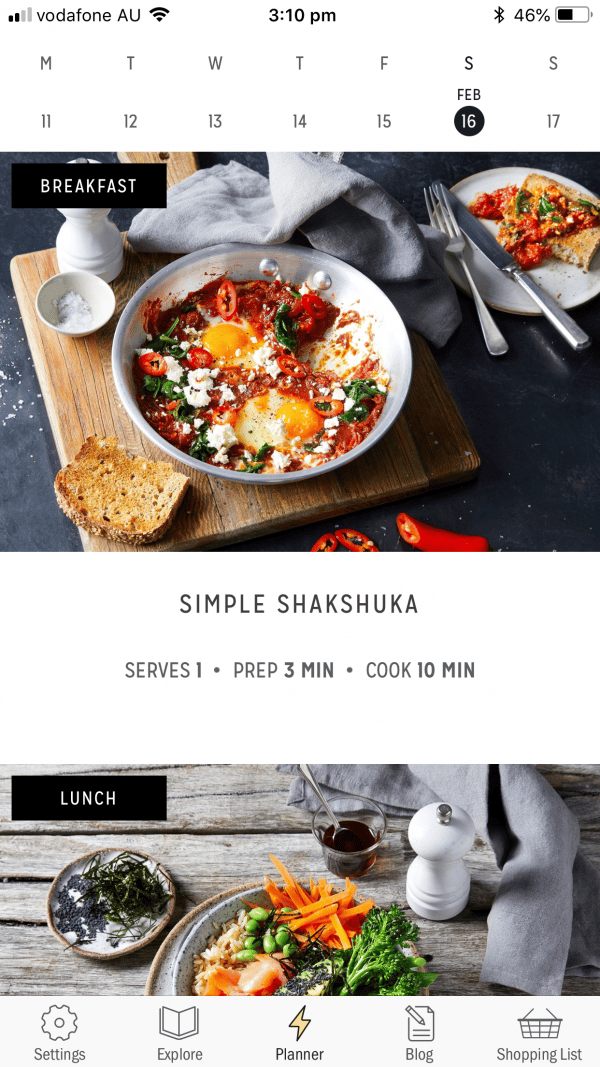This screenshot is from a smartphone, displaying various interface elements and a meal planning app. 

At the top left, there are service bars with the label "Vodafone AU," followed by a full Wi-Fi signal icon in the middle. The time displayed is "3:10 PM." On the right side, icons for Bluetooth (with low signal) and the battery status (at 46%, roughly half full) are visible.

The main content shows a weekly calendar, with the dates 11 to 17 laid out horizontally. Above the date 16, there's an abbreviated "FEB" indicating February, and the 16th is highlighted with a black circle. The days of the week are represented by their initials: MTWTFSS (Monday, Tuesday, Wednesday, Thursday, Friday, Saturday, Sunday).

Below the calendar, there's a heading labeled "Breakfast," accompanied by an image of a meal consisting of a bowl with eggs and various vegetables, placed on a cutting board alongside a piece of toast. The meal appears to be part of a meal planner or menu guide. The bowl is metallic, and the food arrangement suggests a well-thought presentation.

Further down, there's text describing the meal: "Simple Shakshuka serves one, prep three minutes, cook ten minutes." This suggests a recipe or a quick meal guide.

Following this section is another heading labeled "Lunch," below which there's an image of a meal containing vegetables, rice, and a small side dip garnished with what looks like dill and possibly chia seeds.

At the bottom of the screen, there's a menu bar with options: "Settings," "Explore," "Planner," "Blog," and "Shopping List." The "Planner" option is currently highlighted, indicating the active screen the user is on.

Overall, the screenshot encapsulates a digital meal planner app, detailing different meal images and recipes for breakfast and lunch, along with relevant quick-access menu options.